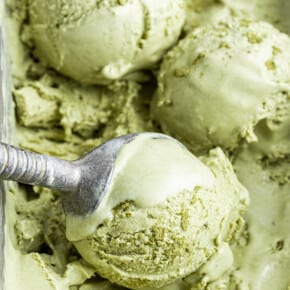A close-up image showcases three scoops of green ice cream, likely pistachio due to its color and the small pistachio bits sprinkled on top. The scene is dominated by a silver ice cream scoop, positioned in the lower left, which is actively scooping a creamy, melting portion of the ice cream, highlighting its decadent and sweet texture. Two other scoops are visible in the background, with one partially cut off at the top of the frame. The ice cream exudes a rich and inviting appearance, with a light source coming from the right, enhancing the creamy texture and myriad of small specks within the ice cream. The scoop itself features a handle with rings for grip, made of sturdy metal, adding to the rustic, artisanal feel of the image.